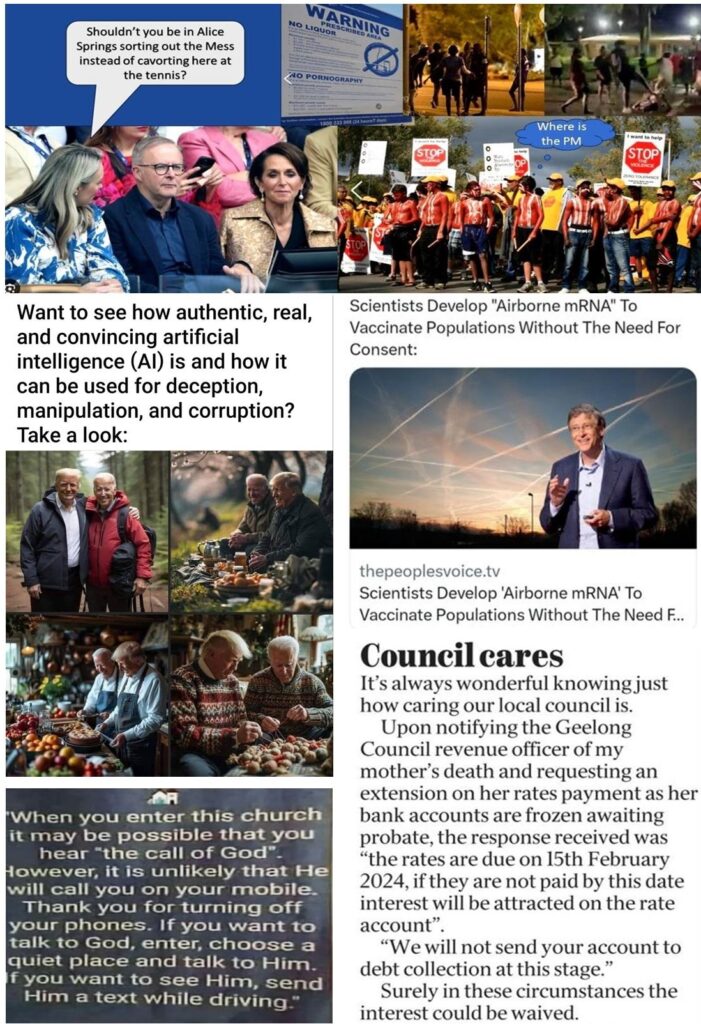A collage of disparate images and text forms an eclectic yet thought-provoking visual narrative. Starting from the top, we see a sequence of images featuring a trio seated in a stadium: a woman, a man, and another woman. The woman on the left, dressed in blue, queries, "Shouldn't you be in Alice Springs sorting out the mess instead of cavorting here at the tennis?" Her gaze is ambiguous, directed either towards the man or the woman beside him.

Adjacent to this, a series of photographs shows construction workers, seemingly in the middle of a strike. The accompanying blue text bubble inquires, "Where is the PM?" Further images depict groups of people clad in black, engaging in chaotic activities on urban streets under the cover of night.

Beneath these are four images that merge reality and fiction—a surreal montage of Trump and Biden with their arms around each other, engaged in various friendly activities like picnicking, crafting Christmas ornaments, and visiting a farmer's market. Above these images, a warning reads: "Want to see how authentic, real, and convincing artificial intelligence (AI) is and how it can be used for deception, manipulation, and corruption? Take a look."

To the left of these contrasting depictions is a humorous yet poignant church sign: "When you enter this church, it may be possible that you hear the call of God. However, it is unlikely that he will call you on your mobile. Thank you for turning off your phones. If you want to talk to God, enter, choose a quiet place, and talk to him. If you want to see him, send him a text while driving."

On the right, an article features a prominent figure from Microsoft—presumably Steve Jobs, despite the mix-up in identification. The headline intriguingly announces, "Scientists develop airborne mRNA to vaccinate populations without the need of..." followed by a reference to a segment titled "Council Cares."

Each element in this collage contributes to a larger commentary on modern technology, social unrest, the potential for AI misuse, and human spirituality, all interwoven in an intricate tapestry.